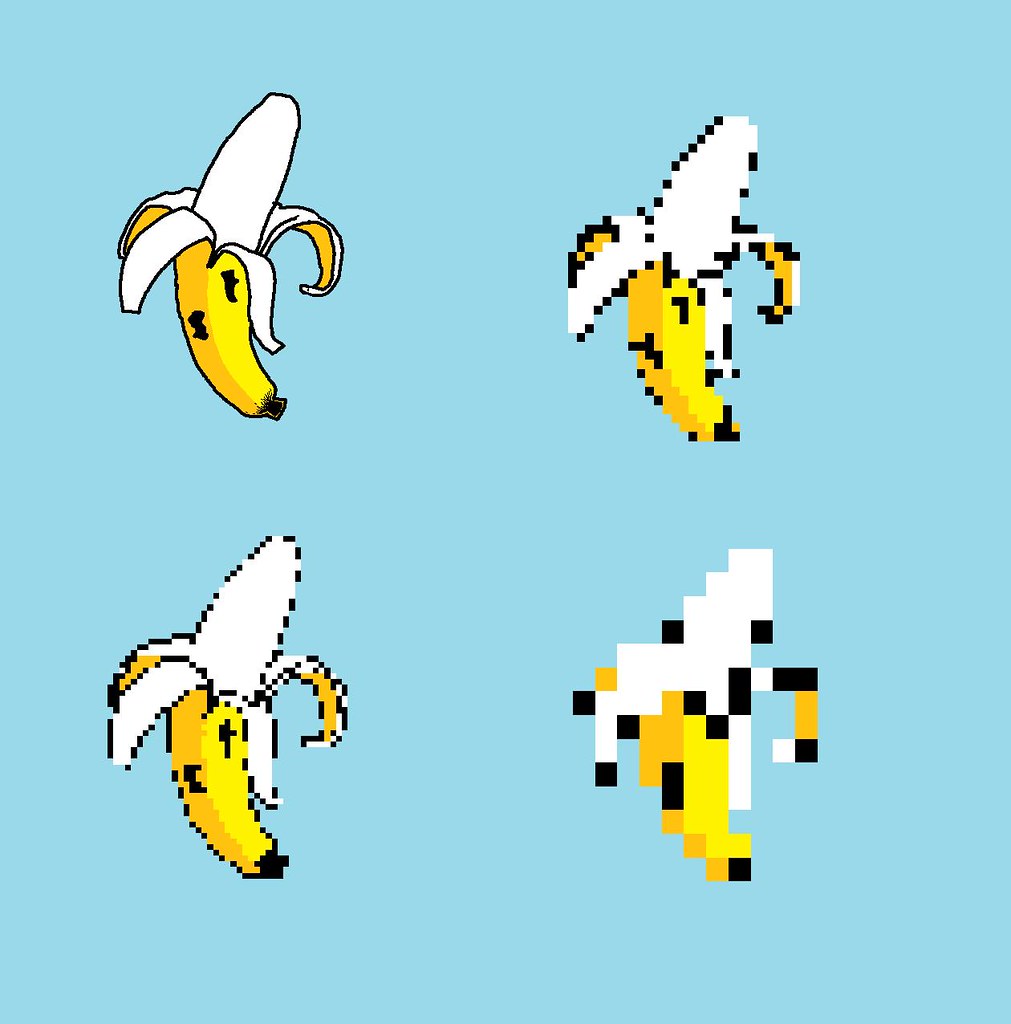The image is a digital artwork featuring four progressively pixelated bananas arranged in a 2x2 grid against a light blue background. The banana in the top left corner is a clean, clear graphic design with a yellow peel, slightly opened to reveal the white fruit inside, and marked by two small black spots. The banana on the top right is more pixelated, with visible square blocks distorting its appearance. The bottom left banana shows increased pixelation, making the image grainier with smaller black squares interrupting the yellow and white colors. Finally, the banana in the bottom right corner is highly pixelated to the point of near indecipherability, appearing as a collection of disjointed colored blocks, barely recognizable as a banana.